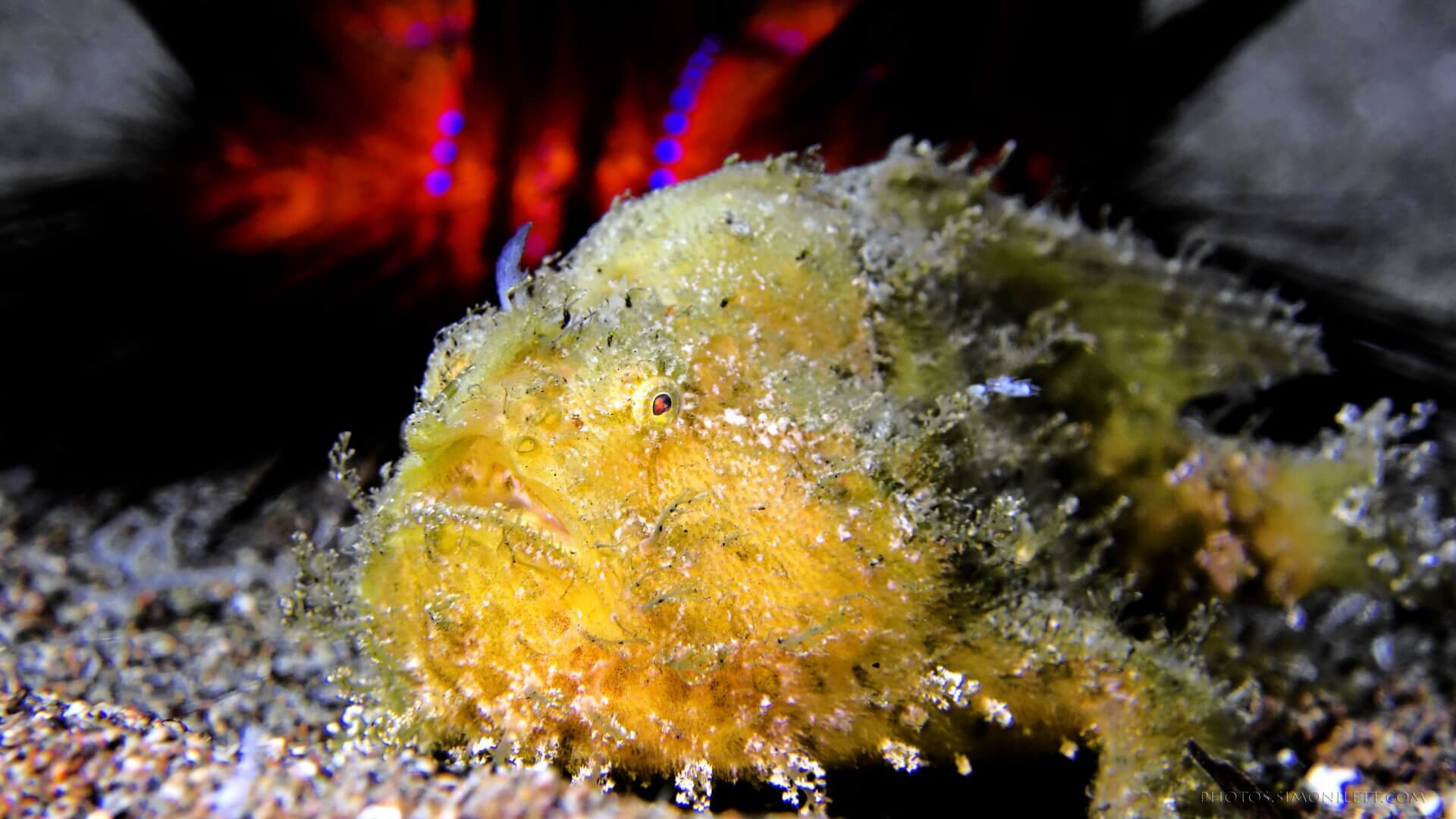The image depicts a unique fish at the bottom of the ocean, blending seamlessly into its environment. The fish has a bulbous face, yellow eyes with black and red centers, and a spiny, rough texture reminiscent of corals, with a dull green overlay that gives it an algae-covered appearance. Its translucent, jelly-like, crystallized surface adds to its camouflaged, almost frost-covered look. The body of the fish is predominantly yellow, featuring black markings and an olive-green dorsal fin. The background showcases a bed of tiny pebbles or ocean debris in shades of brown, beige, black, and white, alongside a gray sea rock wall. There is also a faint, distant red illumination with blue circular designs, possibly hinting at another creature or underwater lighting. Overall, this fish's appearance strikingly resembles its coral surroundings, almost as if it were part of the ocean floor itself.